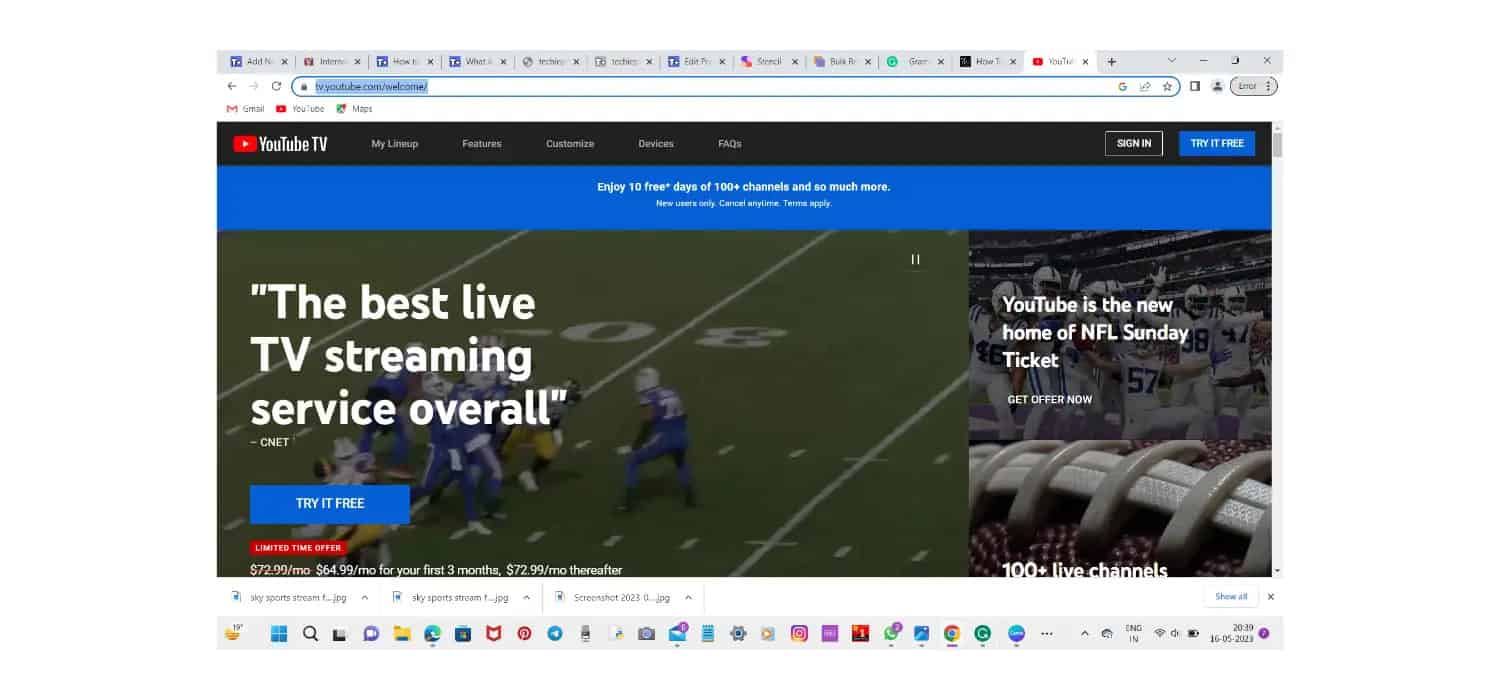In this image, we see a screenshot of a computer screen displaying the YouTube TV website. The view is somewhat zoomed out but still reveals several key elements. At the top, there are approximately ten open tabs, all set against a grey background. Below this, the URL bar indicates YouTube and is highlighted in a light bluish-gray color.

The main content area underneath features a dual-toned background. On the left, set against a black background, the bold text reads "YouTube TV". Adjacent to this are five categories that lead to various sections of the site, followed by options to "Sign In" and a blue "Try it Free" button.

A prominent blue banner below promotes a special offer that reads, "Enjoy 10 free days of 100+ channels and so much more," accompanied by a smaller white sentence beneath it. To the left, the text asserts, "The best live TV streaming service overall."

The background features a live football game, focusing on the field around the 30-yard line, with another "Try it Free" button in white text on a blue background at the lower left.

On the right-hand side of the screen, there is an image of a football team, likely the Dallas Cowboys, celebrating in the end zone. This section also has a notice that "YouTube is the new home of NFL Sunday Ticket."

At the very bottom of the screen, various computer icons are visible, extending from left to right, suggesting this screenshot was captured from a user's desktop.